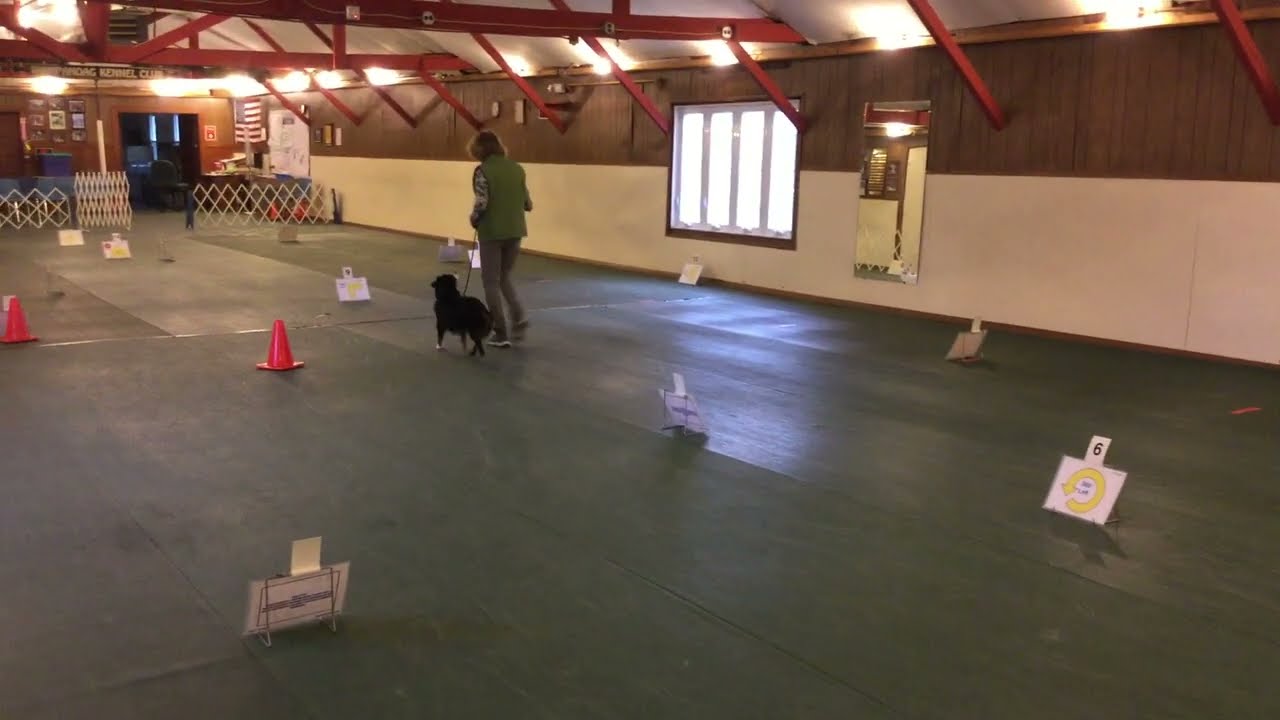In this indoor training facility, a woman is captured mid-walk, training her medium-sized, fluffy black dog. The woman, dressed in a green vest, gray pants, and stylish shoes, commands her dog’s attention as they maneuver through a numbered agility course. The room, likely a large warehouse or community center, features a gray concrete floor scattered with orange cones and various numbered signs, the most visible being number six. The walls of the room are two-toned, with a brown upper half and a lighter tan bottom half, intersected by a window with four vertical glass panes and an adjacent mirror. Red metal support beams stretch from the walls to the ceiling, adding to the structured layout of the space. An American flag adorns one corner while an open window allows a glimpse outside, contributing to the overall dynamic ambiance of the training environment.